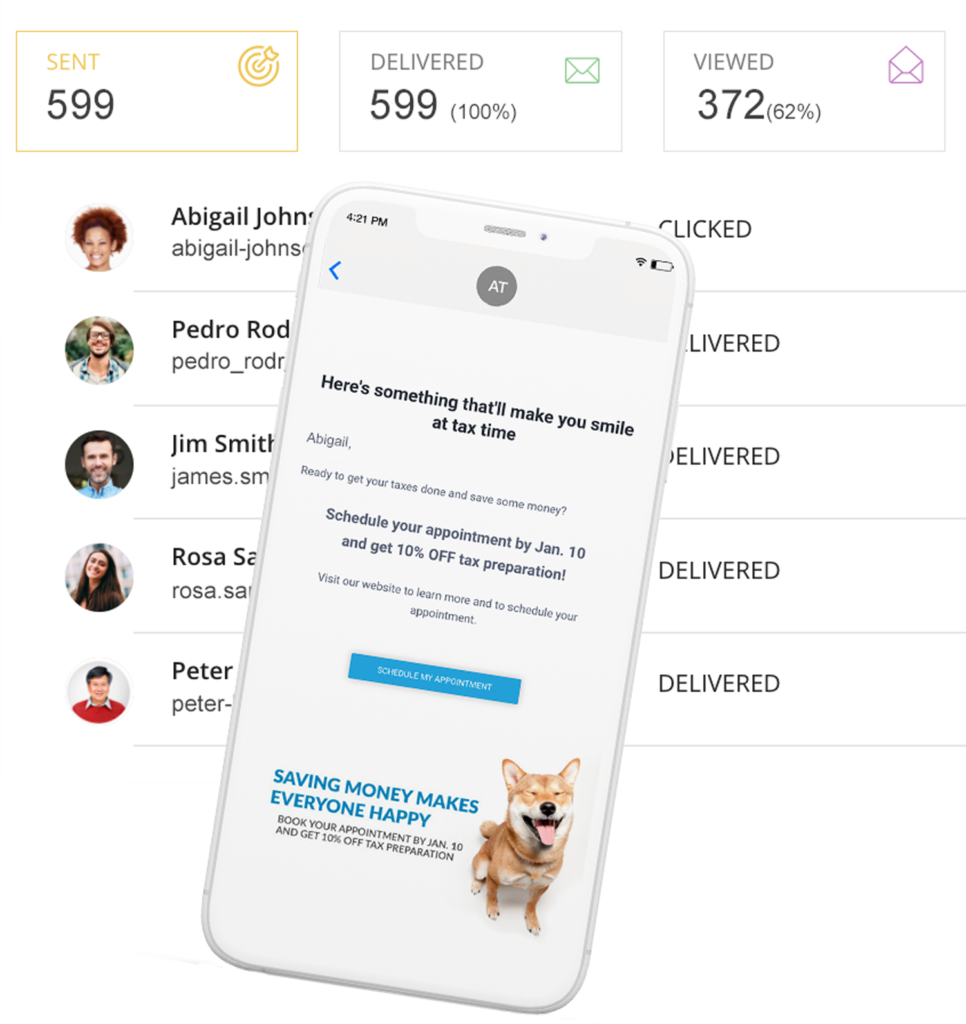The image showcases a computer screen displaying a summary of message send metrics at the top, organized into three columns. The first column is outlined in gold and titled "Sent," indicating the number 599. The middle column reads "Delivered," showing "599 (100%)." The third column is labeled "Viewed" with the statistic "372 (62%)."

Below these metrics, the screen displays a list of individuals lined up in columns, featuring their profile pictures on the left and their names immediately next to them. The detailed list includes a woman, followed by three men, and ending with another woman.

Superimposed on top of this screen is an image of a smartphone, obscuring part of the information beneath it. The smartphone has a white background and displays a message with several key details:
- At the top, the time reads "4:21 PM."
- A gray circle with white letters "AT" is centered on the screen.
- Below it, in black text: "Here's something that'll make you smile at tax time."
- In gray text: "Abigail, ready to get your taxes done and save some money? Schedule your appointment by January 10 and get 10% off tax preparation. Visit our website to learn more and to schedule your appointment."
- A blue button labeled "Schedule Appointment."
- Additional black text at the bottom reads: "Saving money makes everyone happy. Book your appointment by Jan 10 and get 10% off tax preparation."
  
In the lower-right corner of the phone image, there is a cheerful dog with its mouth open, adding a touch of whimsy to the otherwise functional display.